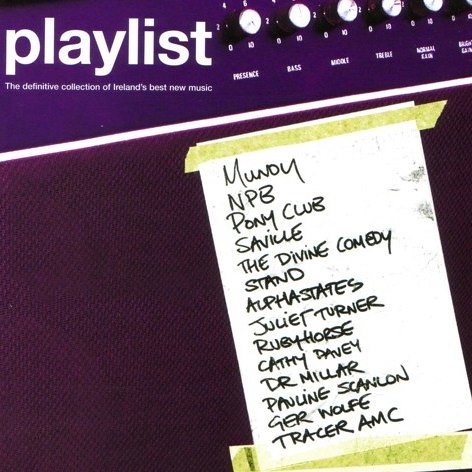The image titled "Playlist" showcases a speaker-like layout with a distinctive music-themed design. At the top left corner, against a lighter purple background, the title "Playlist" is prominently displayed in white text. Beneath this title in smaller print, it reads "The definitive collection of Ireland's best new music."

The upper section of the image features five control knobs labeled "Presence," "Bass," "Middle," and other fading labels, evoking the appearance of an amplifier. Below the knobs is a dark red surface, simulating the speaker's fabric. Taped onto this surface is a piece of white paper secured with yellow tape at the top and bottom. The paper lists various artists' names in what appears to be handwritten text: Mundy, NPP, Pony Club, Saphine, The Divine Comedy, Stand, Alva Stace, Juliet Turner, Ruby Horse, Cathy Davey, Mr. Himmler, Pauline Scandal, Jura Booth, and Tracer AMC. The overall layout and textures suggest a homage to musical equipment, blending elements of sound and artistry.